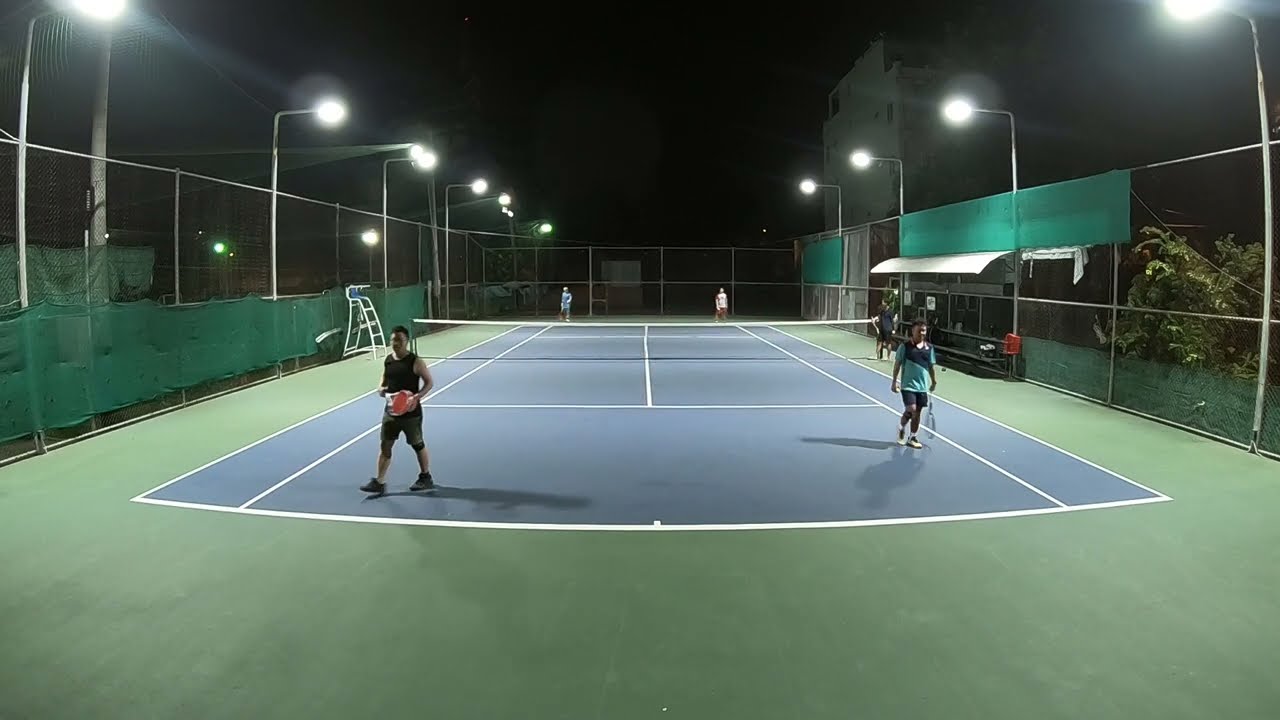This nighttime image captures a doubles tennis match on a well-lit, fenced-in tennis court. The court's inbounds area is a striking blue, outlined with standard white boundary lines, while the out-of-bounds region is green. Tall fence panels surround the entire area, and between each, or every other panel, there are L-shaped poles with white lights illuminating the court.

On the near side of the court, two male players are walking toward the camera. The player on the right wears a teal and blue shirt, blue shorts, and light-colored sneakers, and holds a tennis racket. The player on the left, dressed in a black tank top, dark shorts, and black shoes, holds a red ball. There is also what appears to be an unoccupied judge’s ladder near some benches, suggesting an informal game. 

In the distant part of the court, two additional players, their identities less discernible, continue the match. This immersive, wide-angle view emphasizes the detailed setup and activity of a recreational tennis game under the evening lights.